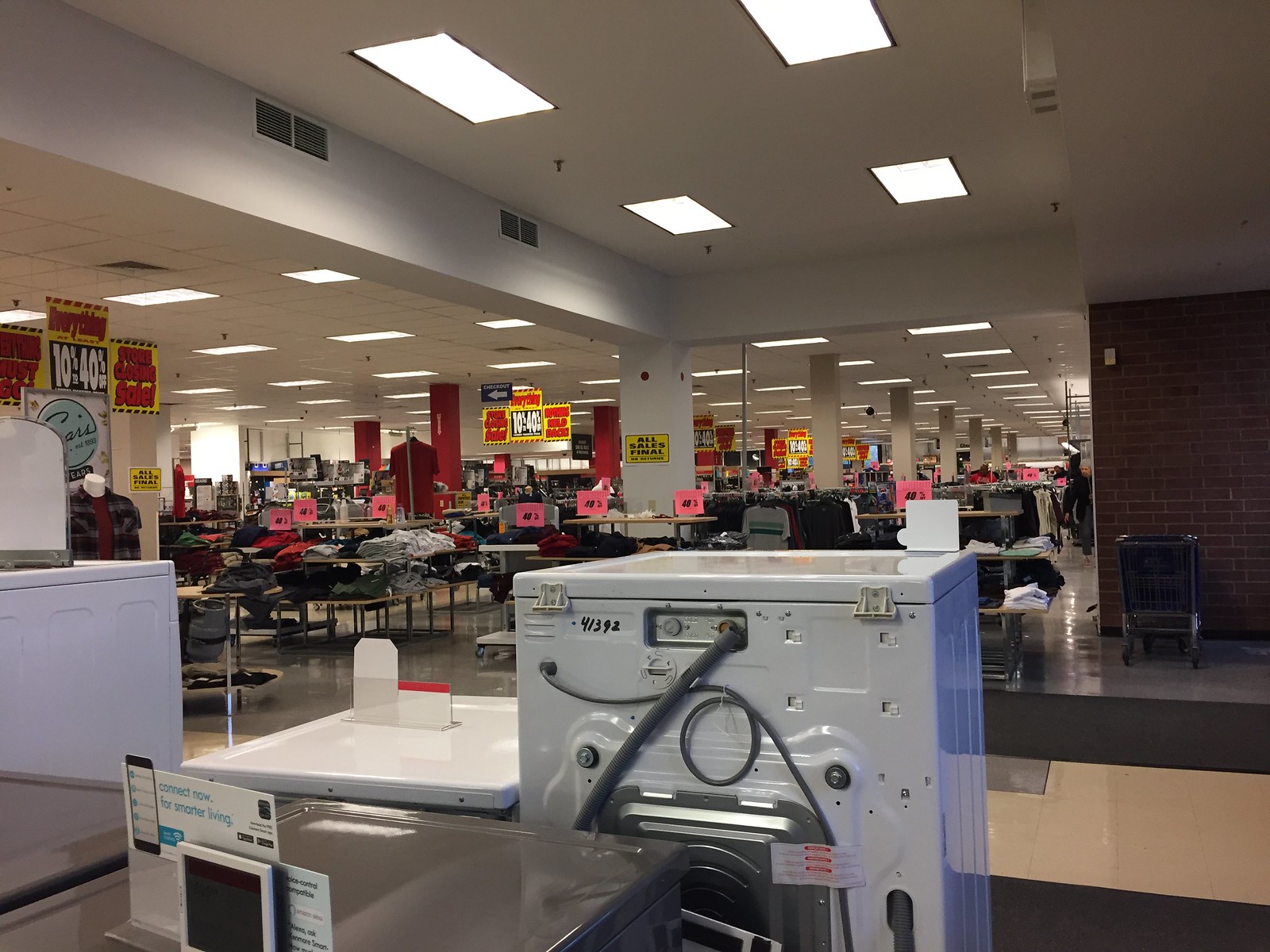The photograph captures the interior of a retail store undergoing a closing sale. In the foreground, there is the back of an indistinct white appliance, flanked by several other white appliances and a dark gray appliance positioned in the bottom left corner. Toward the middle ground, a series of freestanding shelves are neatly stocked with folded clothes, adding to the display. Scattered throughout the store are prominent yellow signs with red writing declaring "Store Closing Sale" and "Everything Must Go." Additionally, a black panel with white text advertises discounts ranging from 10% to 40% off. A yellow sign with black lettering on one of the walls sternly advises customers that "All Sales Final."